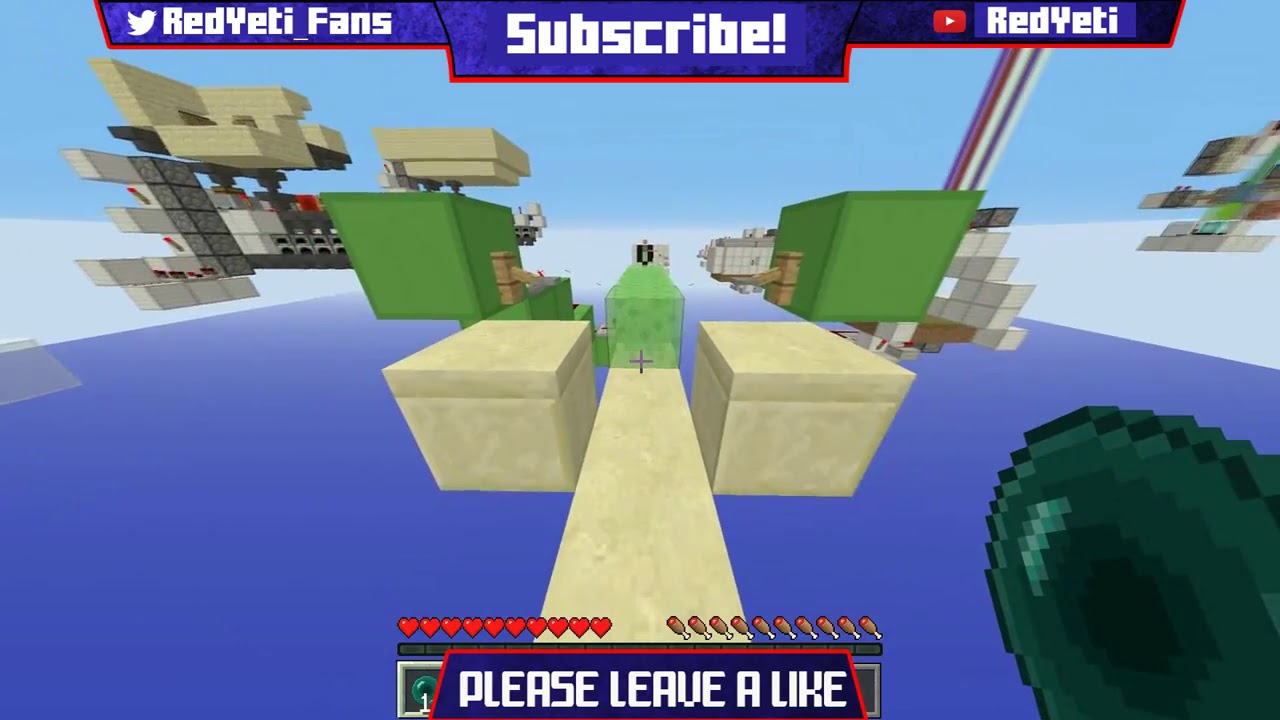This is a detailed screenshot from the popular video game Minecraft, showcasing a YouTube channel's video overlay. At the center of the image, a character is navigating a sky-high sandstone walkway flanked by green blocks, resembling a sky base. Below this, a pool of water adds depth to the scene. The top of the image features a promotional banner with alternating blue, red, and white graphics. The left side of the banner displays a white Twitter icon accompanied by the text "Red Yeti fans," while the middle portion urges viewers to "Subscribe!" in bold white text. To the right, a YouTube icon pairs with "Red Yeti" in red typeface. The bottom of the image includes another prompt in all caps: "PLEASE LEAVE A LIKE." The Minecraft interface is visible with red hearts on the left and drumsticks on the right, indicating the character's health and hunger status. The character appears to be holding an Ender Pearl, a green, jewel-like item. The colors throughout the image span blue, gray, white, light blue, purple, red, tan, and green, contributing to the vibrant and engaging aesthetic commonly seen in gaming YouTube content.